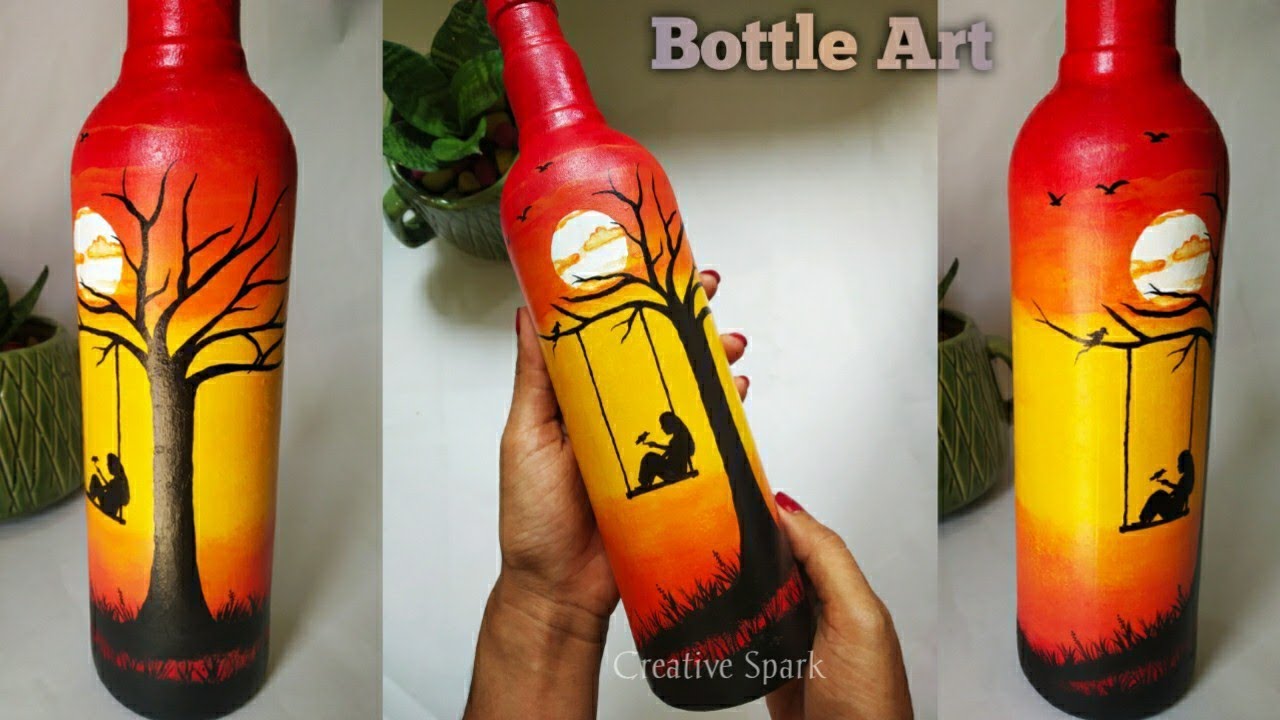The image features a piece of bottle art prominently displayed in a set of three photos. The bottle is intricately painted with a beautiful sunset scene. The top of the bottle is red, transitioning into a striking depiction of a sun setting over a yellow and red-orange horizon. The scene includes a silhouette of a leafless tree, with some grass at its base.

Nestled within the branches of the tree are several birds, and one bird is notably perched on the outstretched hand of a young girl who is seated on a swing. The girl is viewed in profile, her legs lifted gracefully on the swing. The sky also shows birds in flight, adding to the tranquil yet lively atmosphere.

In the first image on the left, the bottle art is shown standing beside a plant, giving it a natural context. The middle image features a pair of hands holding the bottle carefully, again with a plant visible in the top left corner, emphasizing the handcrafted nature of the art. The third image offers a slightly different angle of the bottle, turned towards the left, maintaining the visual continuity with the surrounding plant. These images collectively highlight the detailed craftsmanship and aesthetic appeal of the painted bottle.